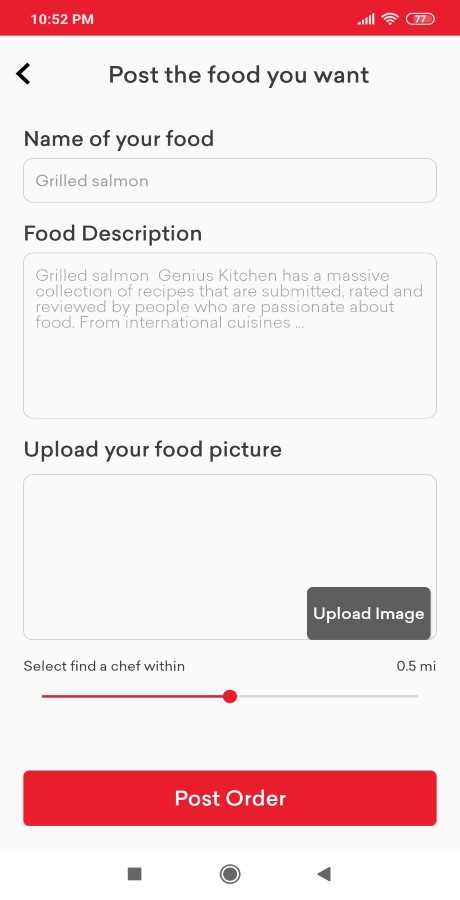In this image, we see a screenshot of an Android device. At the top left corner, the time is displayed as 10:52 PM. Adjacent to the time, the network signal strength bar shows full signal with 5 out of 5 bars, and the Wi-Fi signal strength icon also shows full connectivity at 5 out of 5 bars. The battery indicator displays a charge level of 77%.

The main content of the page includes a text prompt encouraging the user to "post the food you want." Below this, there are fields for entering details about the food: the name "grilled salmon" and the description "grilled salmon."

The text further explains that "Genius Kitchen has a massive collection of recipes that are submitted, rated, and reviewed by people who are passionate about food from international cuisines." There are options to "upload your food picture" and "upload image," followed by a selection to "find a chef within 0.5 miles." Finally, there is a button labeled "Post order."

At the bottom of the screen, the navigation keys of the Android device are visible.